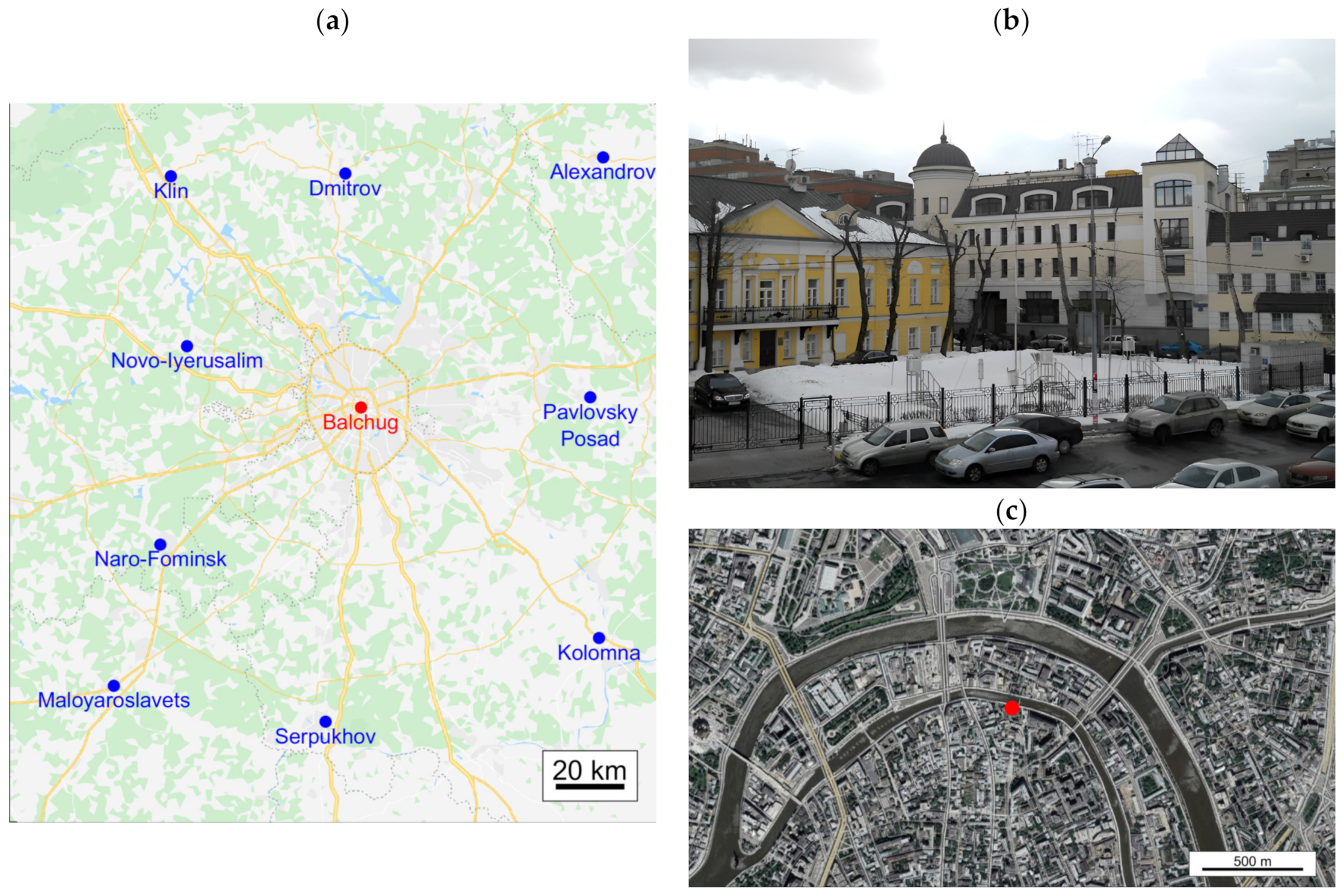The composite image includes three sections labeled A, B, and C. Section A, occupying the left half of the image, features a detailed city map of Balchug, indicated by a red dot. This area is surrounded by a yellow circle, with yellow lines representing roads connecting to nearby towns. The map has green and cream-colored patches, and the towns encircling Balchug are listed in blue: Klin, Dmitriyev, Alexandrov, Pavlovsky Posad, Koloma, Serpukhov, Malo, Iroslavets, Narofominsk, and Novolarizilim. A scale in the bottom right corner indicates distances with a black line marked "20 KM."

On the right side of the image, in the top section labeled B, there is a streetscape showing snow-covered ground, a yellow building on the left, and a white building on the right, with numerous cars and possibly a playground in the foreground. This scene suggests a setting in a Slavic or Germanic region.

Below this, section C features a satellite view map with the letter C above it and a red dot marking a specific location. The satellite map provides a top-down perspective, showing streets, houses, and waterways, with a scale in the bottom corner marked "500 meters."